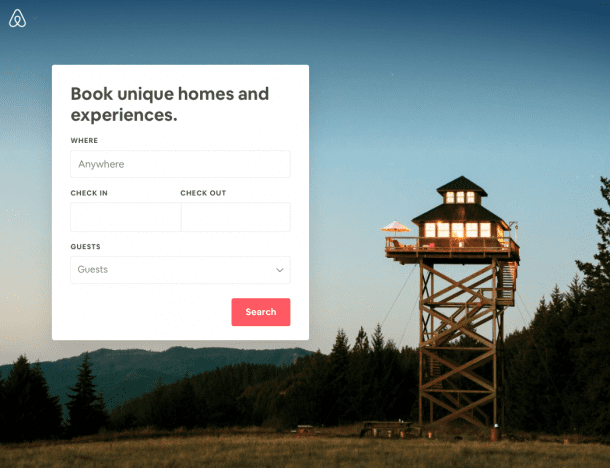The image captures a serene landscape moment, likely taken with a phone, showcasing nature's tranquil beauty. The top of the image features a gradient sky, transitioning from a dark blue at the very top to a light blue, then to a pale white, and finally, a warm hint of yellow, suggesting either a sunrise or sunset. 

Prominently on the right side, there is a quaint little house perched high on a post. This house features a unique dual-roof design and boasts a small balcony around its top. Flanking both sides and filling the center of the scene are tall, dark pine trees that add to the rustic ambiance of the landscape. In the distance on the left, the silhouette of dark mountains or hills provides a dramatic backdrop.

The lower portion of the image is adorned with patches of light yellow and dark green grass, adding depth and texture to the ground.

Overlaying this serene scene, there is an interface for booking unique homes and experiences. On the left, a white box displays black text that reads "Book unique homes and experiences." Below this are various input fields: "Where" with a search bar, "Check in" and "Check out" with respective date fields, and "Guests" with a pull-down menu. At the bottom right corner of this booking interface, there is a prominent red button labeled "Search" in white text.

Overall, the image juxtaposes the peaceful natural setting with a modern-day booking interface, creating a unique and engaging visual experience.